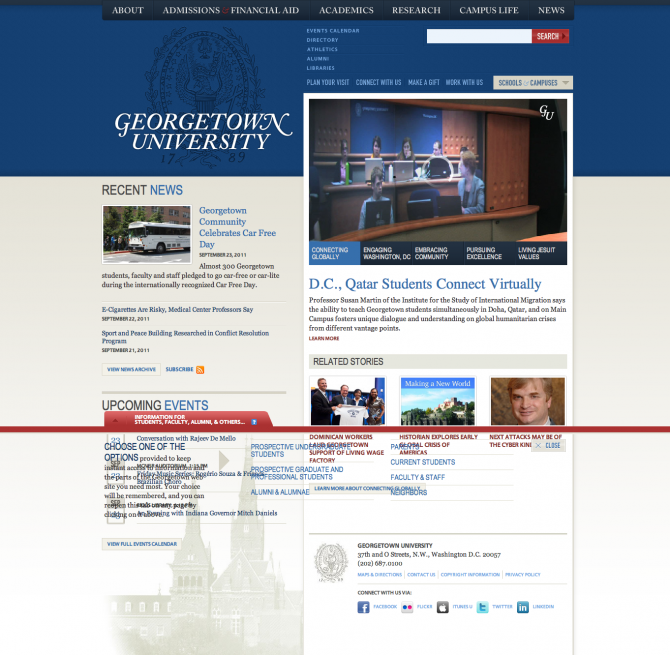The webpage belongs to Georgetown University, presented on a navy blue backdrop. At the top, a blue triangle adorned with the university's black emblem overlaps a navy blue rectangle that stretches across the page. "Georgetown University" is prominently featured in white letters on the left side.

Below, the left panel highlights "Recent News" with the headline "Georgetown Community Celebrates Car-Free Day." Accompanying the headline is an image of a bus picking up a group of students waiting in line. A brief paragraph below the image—a bit too small to decipher—offers further details. Two blue lines with indistinct dates punctuate this section.

A red tab protruding from a red line marks the "Upcoming Events" section. Beneath the tab is a comprehensive list of events scheduled at Georgetown University.

On the right, a photograph depicts a group of seven students engaged in a virtual connection, part of an article titled "DC and Qatar Students Connect Virtually." Further down, a "Related Stories" section features three additional photos, tying into the overarching narrative of the page.